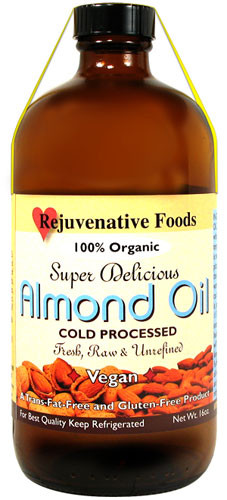This is a detailed photograph of a small brown-colored bottle of almond oil, isolated on a white background for enhanced focus. The bottle features a short black plastic screw-top lid, which is partially covered by what appears to be a yellow seal or band that wraps over the cap and extends downwards. The label on the bottle is predominantly a light yellow color and prominently displays the logo "Rejuvenative Foods." Below the logo, the text reads "100% Organic," "Super Delicious," "Cold-Pressed," "Fresh," "Raw," and "Unrefined." In large white text, it is marked "Vegan," indicating that the contents are suitable for vegans. Additionally, the label features a blue font with a black shadow effect for the text "almond oil," along with an image of several individual almonds at the bottom. Other information on the label includes a directive to keep the product refrigerated, its net weight, and an indication that it is "gluten-free."